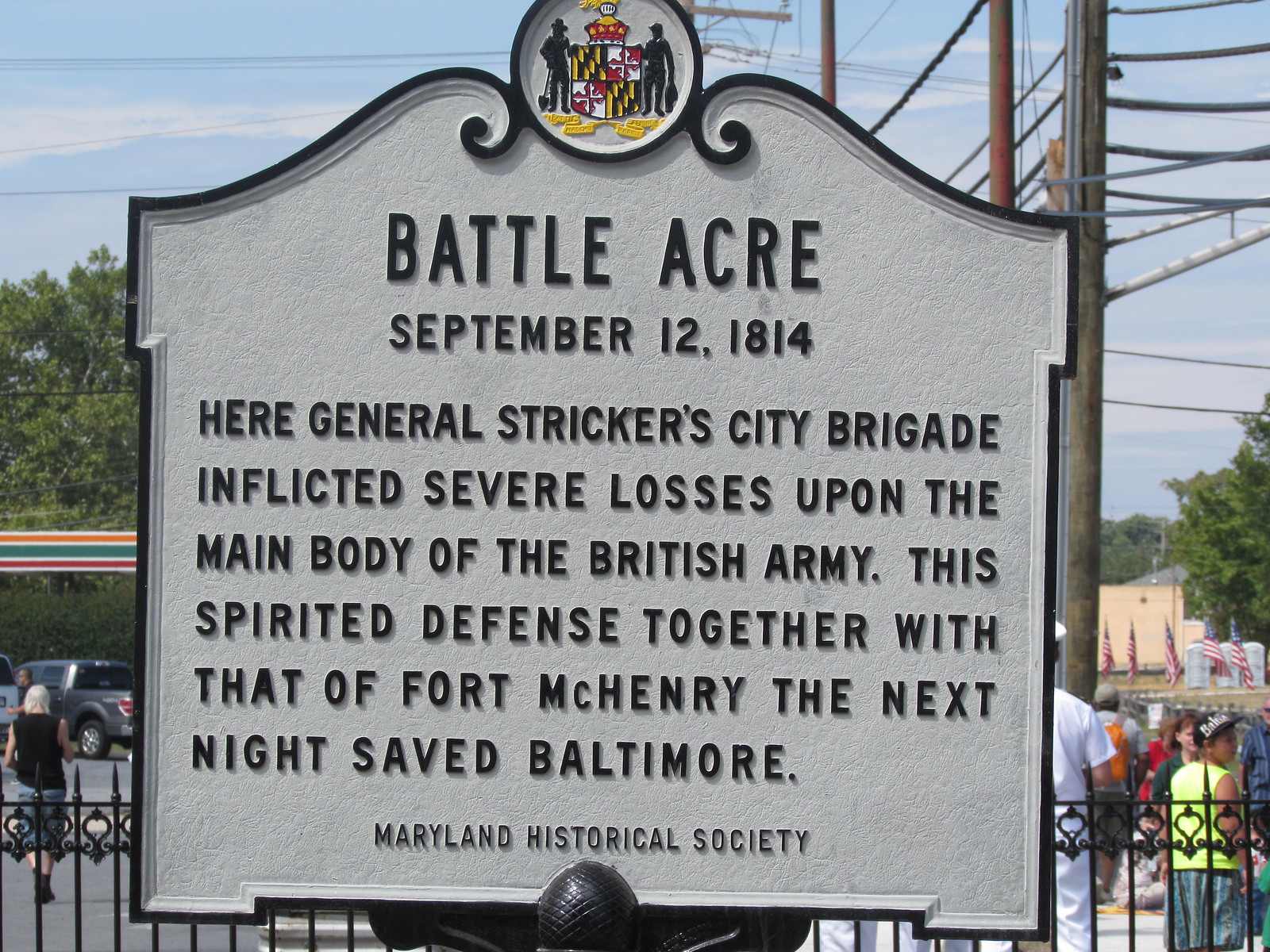This close-up photograph captures a well-maintained metal plaque, prominently featuring a heritage emblem at the top that includes a colored shield flanked by figures on either side. This plaque, with black raised print on a white background, is from the Maryland Historical Society. It is placed at the historical site of Battle Acre, commemorating the battle on September 12, 1814, where General Stricker's City Brigade inflicted severe losses upon the main body of the British Army. The inscription on the plaque reads: "Here General Stricker's City Brigade inflicted severe losses upon the main body of the British Army. This spirited defense, together with that of Fort McHenry the next night, saved Baltimore." The scene behind the plaque features people walking, American flags, and a 7-Eleven store with its signature colors, along with some vehicles and other buildings.